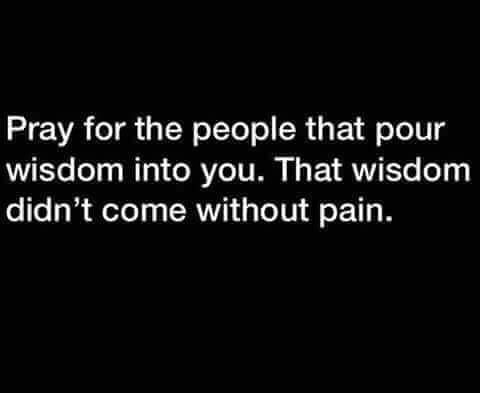This square image features a completely black background with three lines of white text. The text, centered but slightly raised above the middle of the image, reads: "Pray for the people that pour wisdom into you. That wisdom didn't come without pain." The negative space around the text is unequal, with slightly more space at the bottom than at the top. The text is aligned on the left, and the overall design is minimalistic, with no other elements or attribution in the image.